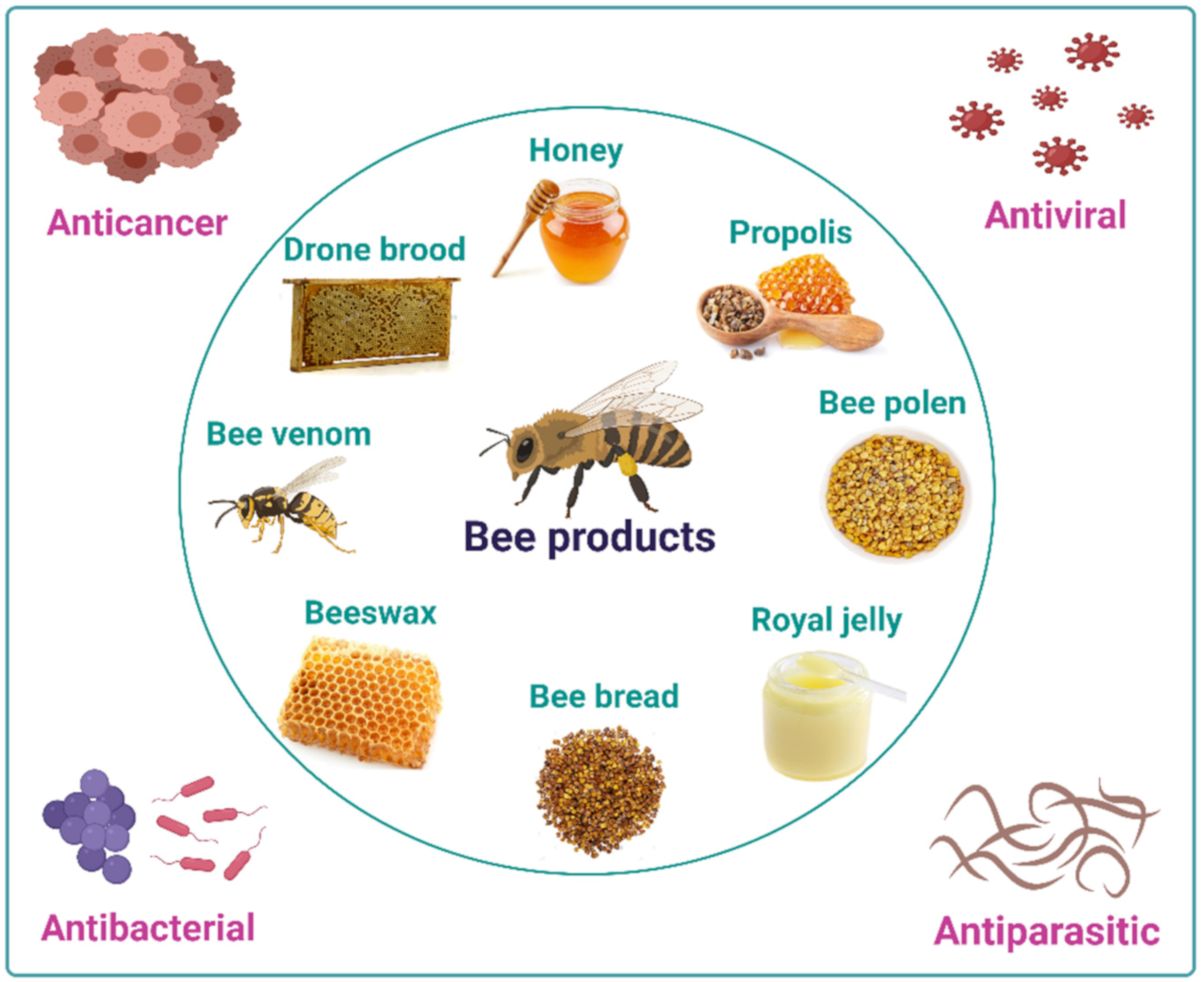The image is a detailed illustration showcasing the benefits of bee products. At its center is a prominently drawn bee in shades of brown and yellow, with the label "bee products" beneath it. Surrounding the bee, within a thin light green turquoise circular border, are various bee-related products positioned like a clock. Starting from the top and moving clockwise, these products include honey (depicted in a jar), propolis (illustrated with a honeycomb and a spoon), bee pollen (shown in a bowl), royal jelly (depicted as a light yellow substance in a bottle), bee bread, beeswax, bee venom, and drone brood.

At each of the four corners of the image, additional illustrations link specific health benefits to these bee products. The top left corner, labeled "anti-cancer," features pink colored cells with darker pink nuclei. The top right corner, labeled "antiviral," displays red circular forms with spiky protrusions. The bottom right corner, labeled "anti-parasitic," includes brown squiggly shapes representing parasites. The bottom left corner, labeled "antibacterial," shows clusters of purple circles and pinkish rounded rectangles with tails. The entire composition is set against an all-white background, creating a clear and informative visual representation of the diverse benefits and types of bee products.